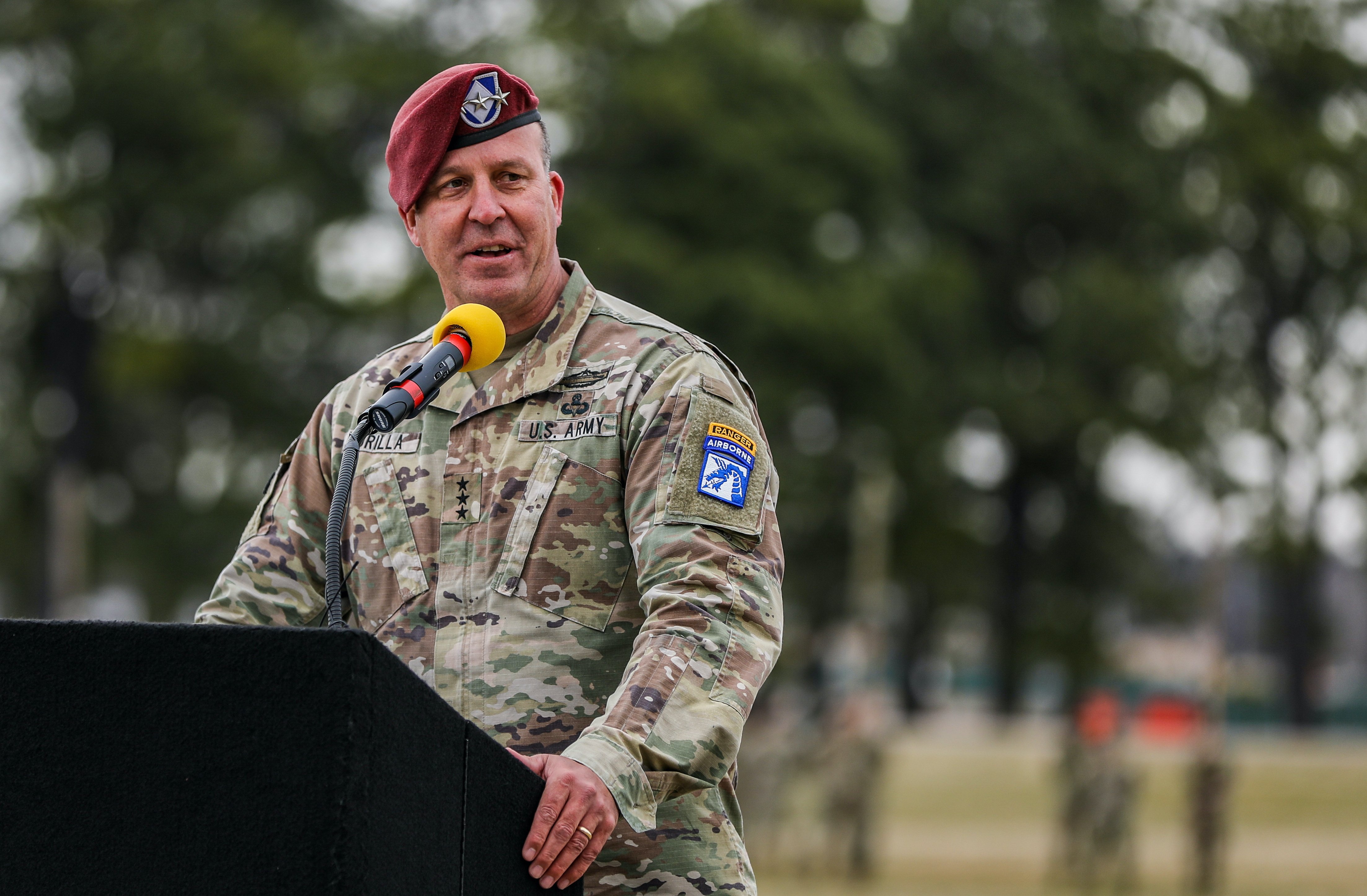The photograph captures a male, likely a U.S. Army officer, standing at a black-topped podium and delivering a speech with a content but serious expression. He is clad in full camouflage fatigues, identified by the label on his left lapel reading "U.S. Army," with multiple patches on his uniform, including a prominent blue patch with a yellow band on top on his left shoulder. The officer wears a gold wedding band on his visible left hand, which is placed on the podium, and his right hand similarly rests nearby. He dons a red beret adorned with a patch at the forehead. The podium features a microphone distinguished by its yellow cover and two red bands. Behind him, the blurred background reveals green foliage, silhouettes of other military members, and a landscape devoid of direct sunlight, suggesting an overcast day. The officer's name partially visible on his uniform reads 'R-I-L-L-A'. Overall, the image conveys a moment of significant address amidst a natural setting.